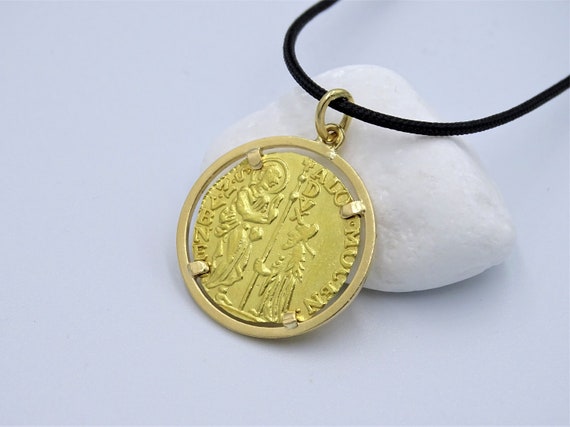The image features a close-up of a medallion necklace displayed against a light off-white or very light blue background. The focal point is a gold, coin-like medallion adorned with two figures facing each other at the center. There is also an inscription on the medallion, though it is hard to decipher; it appears to possibly read "Talomucen" on one side and "S-M-V-E-N-E" on the other. The medallion is secured within a circular clasp and is suspended from a black, round cord that resembles a thick shoelace. This cord runs through a small ring atop the medallion, making it suitable for wearing around the neck. The necklace is resting against a painted white rock, which serves as a prop underneath the black cord, giving the scene a staged yet natural display.